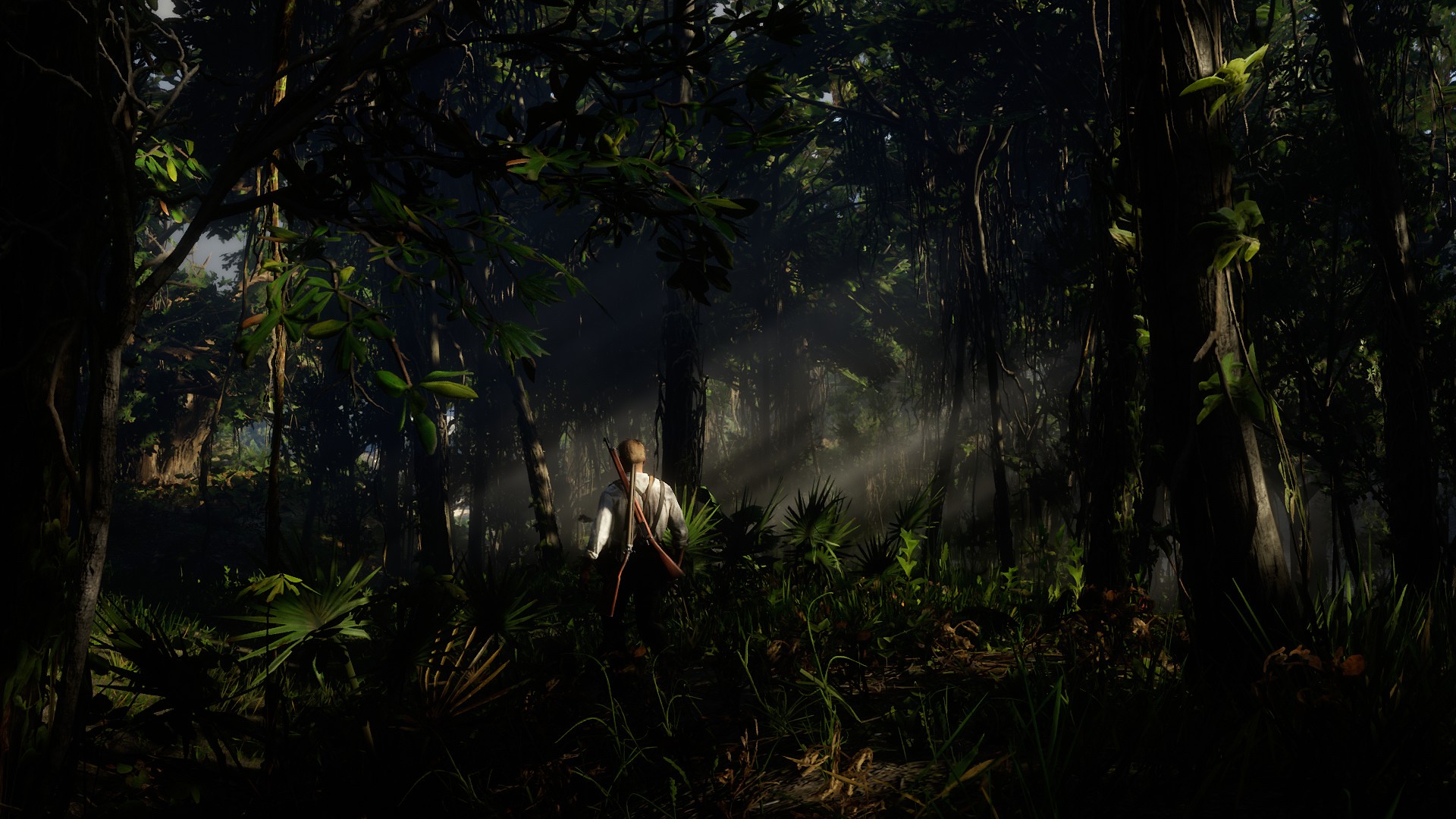In this detailed image, likely captured in a dark, dense forest or a tropical jungle, we see an intricate landscape filled with lush vegetation. The scene is predominantly green and brown, with numerous trees and plants creating a crowded and vibrant environment. Here and there, vines dangle amidst the dense foliage. In the upper left portion of the image, two-thirds of the way up, a patch of gray sky peeks through a small break in the trees. Additionally, faint blue sky is visible through subtle openings, adding to the layered depth of the forest canopy.

At the heart of the image, slightly to the left, stands a lone figure with their back to the viewer. This person, wearing a long-sleeve white shirt and black pants, has short brown hair and appears to be carrying a bow and arrow on their back, possibly attached via a harness. They seem to be trekking further into the dense undergrowth.

To the right of the character, sun rays penetrate the thick canopy, casting "god rays" of light at an angle, some of which sweep dramatically across the scene, creating stark contrasts of light and shadow. Despite these light beams, the overall scene remains quite dark and shadowy, enhancing the sense of depth and the mysterious atmosphere of this wilderness, which might even give the impression of being part of a modern, realistic video game rendering, considering the quality and style of the animation.